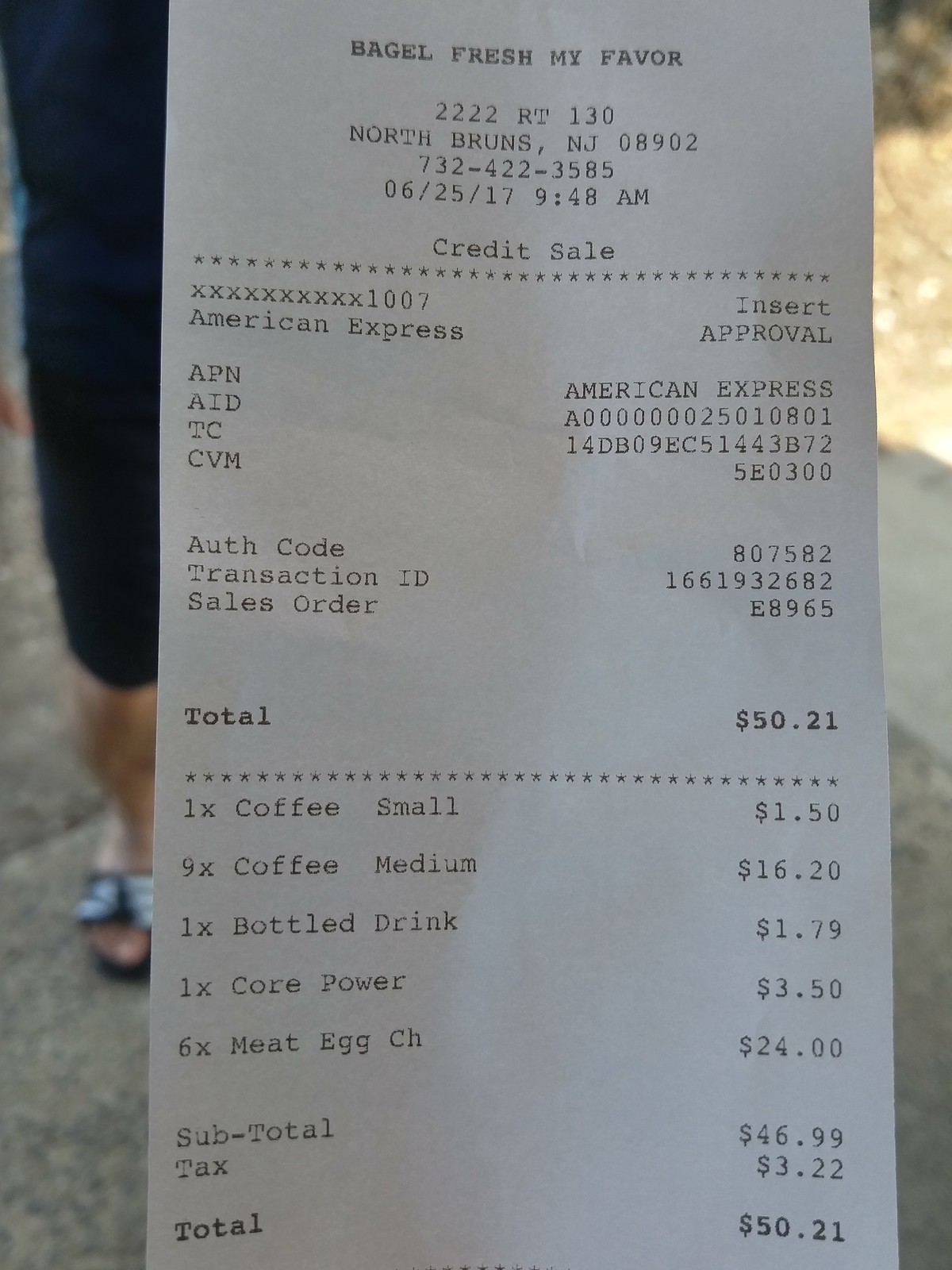This photograph captures a lengthy, rectangular white receipt with black text, prominently displaying the header "Bagel Fresh" at the top. Held out against an outdoor backdrop, the receipt lists an address in New Jersey, including the city, zip code, and phone number. The transaction details reference a date of June 25, 2017, at 9:48 a.m., noting a total amount of $50.21 for a credit sale via American Express, complete with an authorization code and sales order.

In the background, a slightly out-of-focus individual with light skin stands behind the receipt. They are dressed casually in a blue shirt, dark blue capri pants, and black-and-white flip-flops, adding contextual depth to the scene.